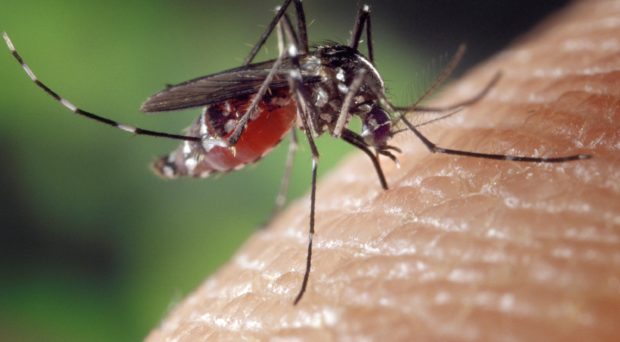This rectangular close-up photograph captures an astonishingly detailed view of a mosquito in the act of biting human skin. The image is dominated by the mosquito, revealing every intricate feature of its body. The mosquito’s stinger is angled eastward, while the tail end of its body points west. The mosquito itself is primarily black with subtle white stripes and sports a distinctly red or pinkish-salmon colored abdomen, likely swollen from the act of feeding. Its multiple delicate legs spread out from its tiny torso, securing its position on the fair, Caucasian skin, which appears magnified, showing every tiny pore and texture. The mosquito’s almost translucent wing, also black, is slightly visible, adding a layer of fragility to its otherwise robust structure. The striking contrast between the mosquito and the pale skin underscores the creature’s minute yet impactful presence in the natural world.